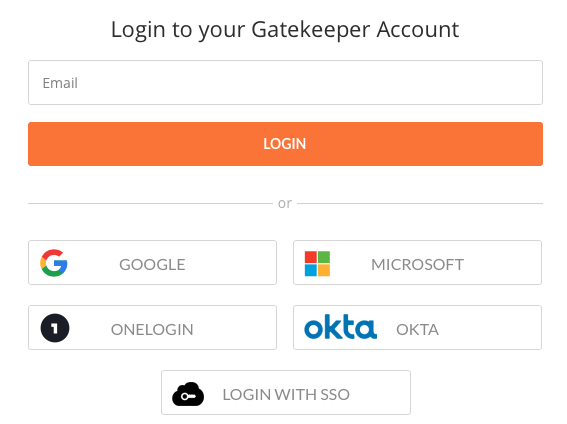Screenshot of a login page for a Gatekeeper account. At the top, the page header reads, "Login to your Gatekeeper account." Below this, there is a text box labeled "Email" for entering an email address. Centrally placed on the page is an orange rectangular button with the word "Login" written in white. Beneath this button, the text "OR" appears, followed by options to log in using various services.

The alternative login options include:
1. Google - Represented by the Google icon, a capital "G" composed of red, yellow, green, and blue segments.
2. Microsoft - Depicted with a logo of a square divided into four smaller squares in red, green, blue, and yellow.
3. OneLogin - Illustrated with a black circle containing a white numeral "1."
4. Okta - Displayed in blue lowercase letters "okta."

Next to the option "Login with SSO" is an icon of a black cloud featuring a white key in the center.

The image does not contain any photographic elements, people, animals, birds, plants, flowers, trees, buildings, automobiles, or airplanes.